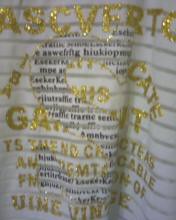A small, vertically oriented image depicts what appears to be a textile sign with a slightly rectangular shape. The central focus of the sign is an outlined 'S' rendered in black lettering. Overlaid on this outline are various words, applied in a striking gold glitter. These words are positioned at unique angles, creating a dynamic and visually interesting effect, though they are challenging to decipher due to the glittering texture. The overall composition combines the elegance of the glitter with the boldness of the black 'S,' offering an intriguing interplay of colors and forms.